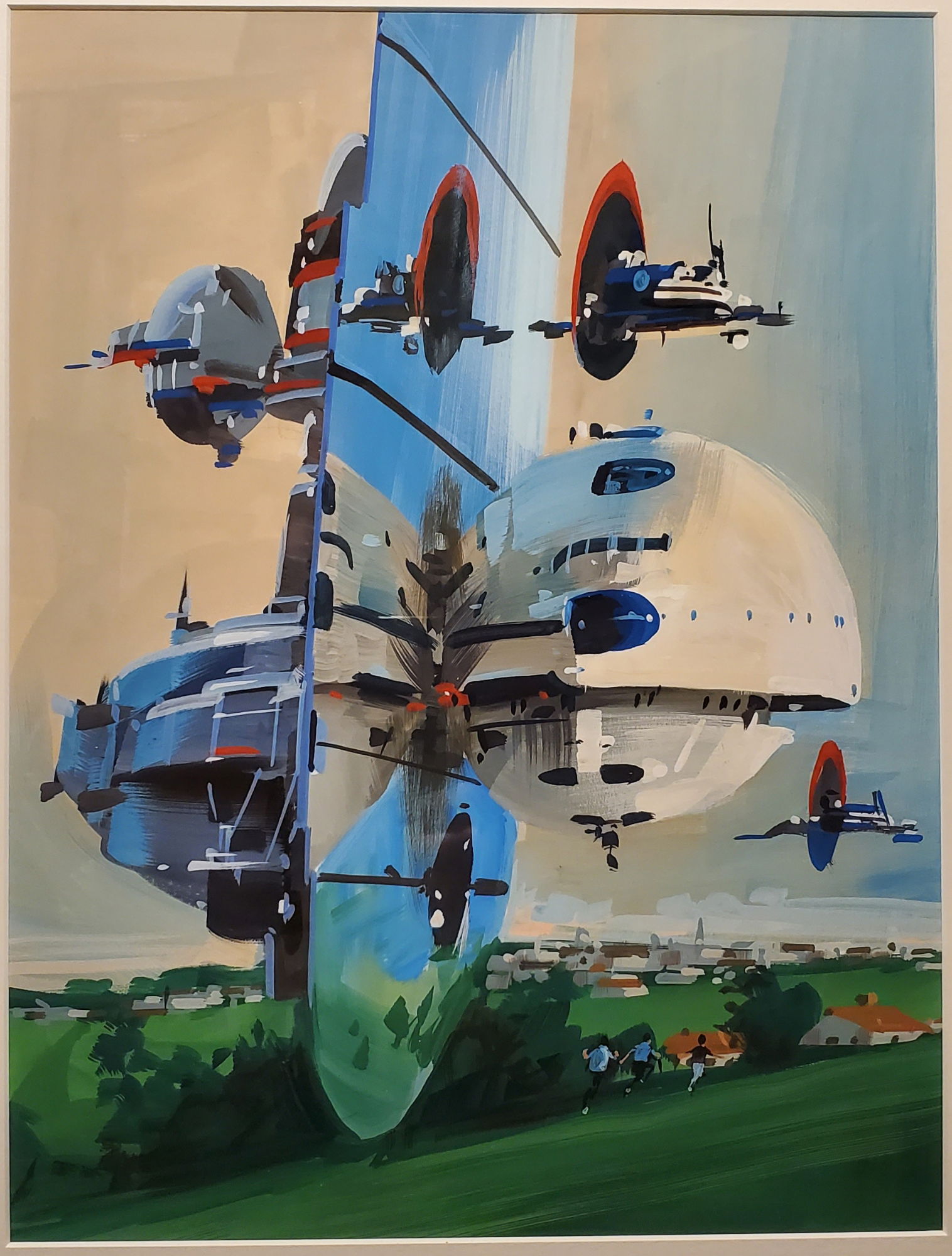In this vivid painting, a large spaceship teeters on the brink of landing, its imposing central fin gleaming with a reflective sheen. Atop the fin, two articulated arms extend outward, fostering a sense of mechanical complexity. On the left, a cylindrical, gray extension adorned with red stripes juts out, while on the right, a smaller, water ski-shaped spacecraft seems to be emerging.

Further down, a sizable, white globe-like structure clings to the spaceship's side, its smooth surface illuminated by a central blue light. Adjacent to this, another broad, gray, rounded segment protrudes from the central fin, adding to the ship's elaborate design. The ground below features a hilly, grassy area dotted with shrubs, into which the fin seamlessly extends.

In the background, a cluster of white houses stands in stark contrast to the spaceship's futuristic aesthetic. On the ground, three figures are captured mid-flight, fleeing the descending craft. Two wear light blue t-shirts and black pants, while the third sports a black shirt and white pants, all with their backs turned in palpable urgency.

Adding to the scene's dynamic tension, a small flying craft, encircled by a striking red ring, hovers on the right side of the image, mirroring the jet ski-like shape of the smaller emerging ship. The overall composition blends elements of terrestrial familiarity with otherworldly intrigue, making for an arresting and richly detailed visual narrative.